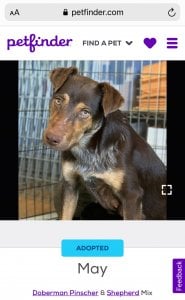This image is a screenshot from the PetFinder website, featuring a predominantly white background. At the top, a long gray search bar stretches nearly the entire width from left to right. On the left side of the search bar, there are two black "A" icons—one smaller and one larger. In the center is a black lock symbol, followed by the text "PetFinder.com" in black letters. To the far right, there's a black refresh button.

Beneath the search bar, on the left, the word "PetFinder" is displayed in purple cursive text. Adjacent to it on the right, the text "FIND A PET" is written in black, all-capital letters, accompanied by a dropdown arrow pointing downward, a purple heart icon, and three purple horizontal lines stacked vertically, each about a quarter inch long.

The main section below this header contains an image framed by black borders on the left and right sides. The image features a brown dog looking directly at the camera with its head slightly tilted down to the right. The dog has a lighter brown stripe down its nose and brown eyes. A cage is visible behind the dog, with a blue wall in the background.

Below the image, a light blue border overlaps the bottom edge. Overlapping both the blue border and the white background beneath it is a blue tab with the word "ADOPTED" written in purple. Beneath this, a white section extends to the bottom of the page, with the word "MAY" in black text.

Further down, the text "Doberman Pinscher" is written in purple with an underline. Following it, "AND SHEPHERD" is displayed in purple, with "MIX" in black text. A purple tab extends upward from the bottom right corner, with "FEEDBACK" written in white letters oriented sideways from bottom to top.